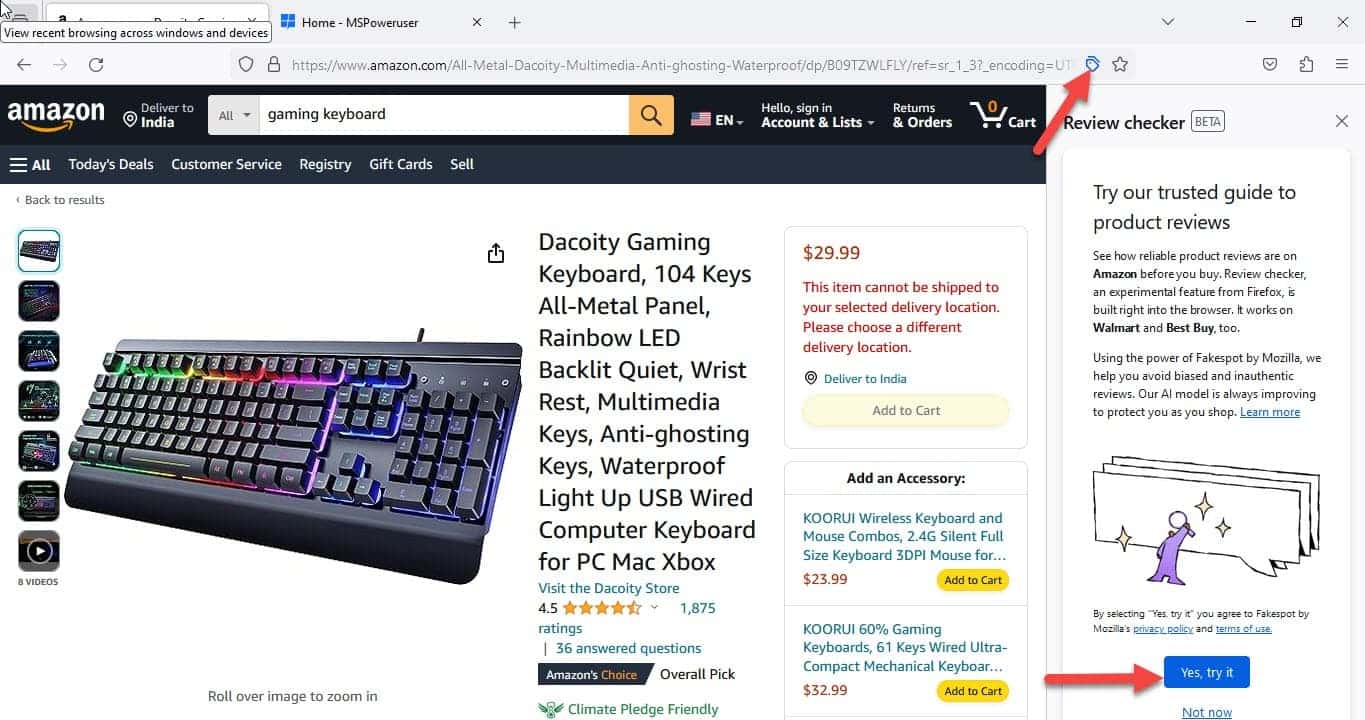This image captures a detailed overview of an Amazon search result page within a web browser, where the user has two open tabs: one for the Amazon search results and another for a Microsoft Power User page. In the Amazon tab, the webpage features the familiar black header, indicating the item will be delivered to the user’s location. The search bar shows the query "gaming keyboard," with a yellow magnifying glass icon next to it. To the right, there's an indicator of the site’s language being English (US), an account sign-in button, links for returns and orders, and a shopping cart icon.

The main focus of the screenshot shows a specific search result that the user has clicked on, displaying a highlighted image of an RGB gaming keyboard from an angled perspective. Located on the left side, there are smaller thumbnails for different views of the product. The keyboard is marketed as the Ducati Gaming Keyboard, featuring 104 keys, an all-metal panel, rainbow LED backlighting, quiet keypresses, and an included wrist rest. To the right of the product description are details such as the price, options to add the item to the cart, and a selection of accessories related to the keyboard.